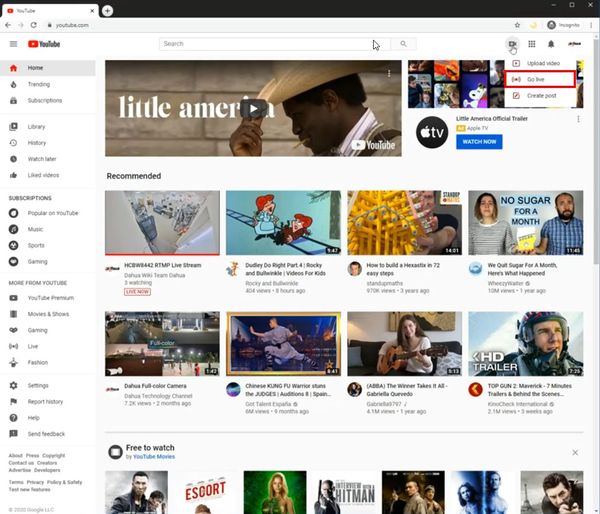This image captures the layout of YouTube's homepage in a comprehensive manner. A black border, approximately an inch in width, frames the top of the page. Prominently displayed on the left side is an expandable tab, which when extended, showcases "YouTube" written in black adjacent to the iconic red YouTube logo. Below this section, a navigation bar includes a left arrow, right arrow, refresh button, and a long search bar with "YouTube.com" inscribed within it.

Directly beneath this, on the left-hand side, there's a sidebar menu featuring three black lines followed by the YouTube red play button and black "YouTube" text. This sidebar lists tabs in a vertical column, including Home, Shopping, Subscriptions, and Library History among others, totaling six main options. Underneath the main options, a section dedicated to Subscriptions showcases four more tabs, followed by a "More from YouTube" segment that lists eight additional tabs.

In the bottom left corner, there is a section providing more information. Adjacent to this, and spanning the top of the page to the right, we see another search bar accompanied by a search icon. Further right, there are four icons arrayed in a horizontal line.

Below the primary search bar, the main content of the homepage starts with a prominent, rectangular video thumbnail of a black man wearing a cowboy hat, facing left. The video is titled "Little America" and includes a play button with a small YouTube logo and white play button in the bottom right corner. To the right of this main thumbnail, there are two smaller video thumbnails.

Underneath this top section, a black circular icon with the Apple emblem followed by "TV" is displayed, flanked by accompanying information. The "Recommended" section begins below this, featuring four video thumbnails in a row with respective details underneath each. Following this pattern, another row of four video thumbnails with corresponding information is present.

Further down, a "Free to Watch" section is highlighted, with an enticing line "Buy YouTube Movies" written in blue lettering. Finally, partially visible, seven movie thumbnails extend horizontally, hinting at additional content available for users.